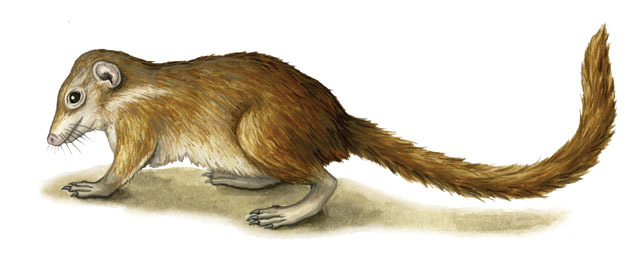This is a detailed, colored pencil-style drawing of a small mammal, resembling a rat or squirrel. The animal, depicted against a white background, is facing left, providing a side profile view. It is predominantly medium brown with a white belly, mouth, and legs. The creature's fur is dense, and it features small ears, prominent whiskers, and a visible dark eye, giving it a somewhat frightened expression. The animal is kneeling on four legs, though only three are visible, and displays long, sharp, black claws. Notably, its tail is extraordinarily long—longer than its body—curving upwards at the end and is also fur-covered. The drawing includes a shaded shadow beneath the animal, adding depth to its appearance.